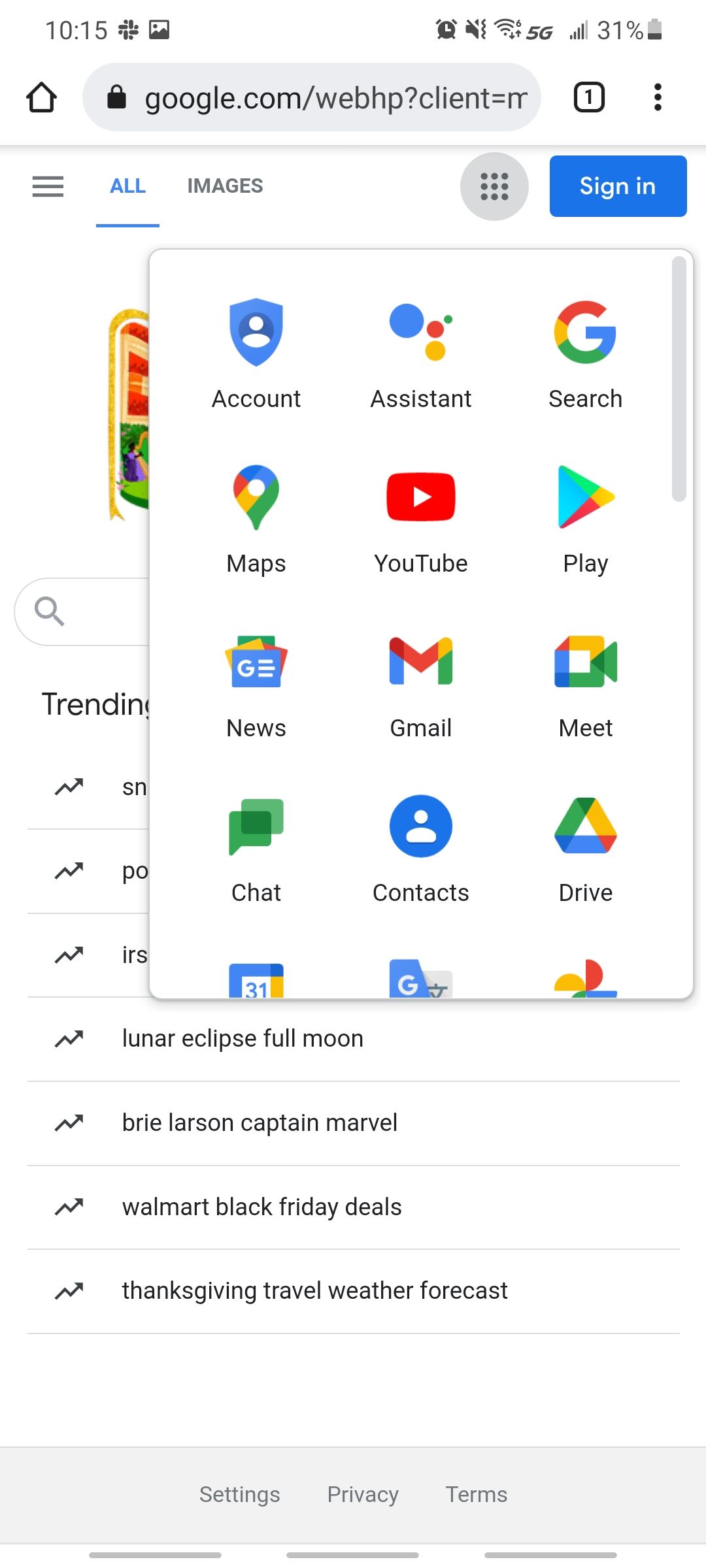A screenshot of a Google search page is displayed. At the top of the screen, the time is shown as 10:15, along with status icons indicating it is connected to 5G and the battery is at 31%. The volume appears to be muted. Below the status bar, the Google logo is prominently displayed on the browser tab, indicating the user is on google.com with one tab open. To the left of the address bar, the home button is visible. To the right, there is a series of three lines (menu button), which is currently selected and highlighted. An adjacent image icon and a 'Sign-in' button are also visible, indicating the user is not signed in.

Beneath this, a grid of app icons is shown, having been accessed by clicking on a three-by-three dot matrix icon representing Google's suite of applications. The apps displayed include: 
- First row: Accounts, Assistant, Search, Maps, YouTube, Play
- Second row: News, Gmail, Meet
- Third row: Chat, Contacts, Drive, along with three additional apps.

Below the grid of apps, part of the Google homepage is visible. A search bar and several trending topics are partially obscured by the apps' dialogue box. Trending topics include "Lunar Eclipse," "Full Moon," "Brie Larson," "Walmart Black Friday deals on Thanksgiving." At the very bottom of the screen, there is a grey bar containing links to "Settings," "Privacy," and "Terms."